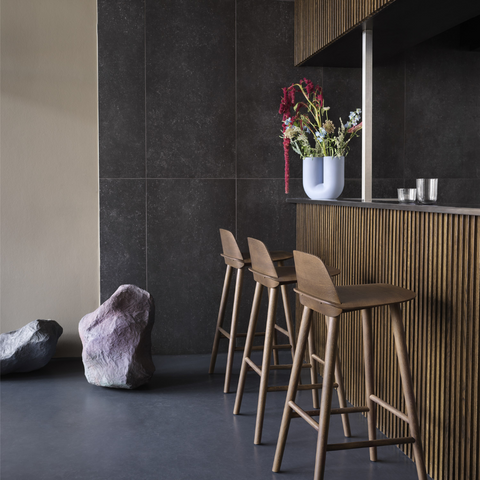The indoor photograph captures the side of a dining area featuring three minimalist, Asian-inspired wooden barstools with short backs. Positioned at a bar, the stools overlook a space accented by vertical wooden slats on both the bar's front and its matching overhang. To the right of the stools sits a countertop adorned with two small glasses, one a short circular cup and the other a whiskey cup. A striking U-shaped white vase filled with purple, pink, and yellow wildflowers, including a distinctive red element, adds a touch of nature to the scene. A single metal pole supports the bar’s overhang. The background reveals a contrast between gray stone panels and a light brown plaster wall, while the floor is made of gray cement. Adding a unique decorative touch, two large boulders—one a light violet hue and the other shiny black—are situated behind the last stool to the left of the bar.